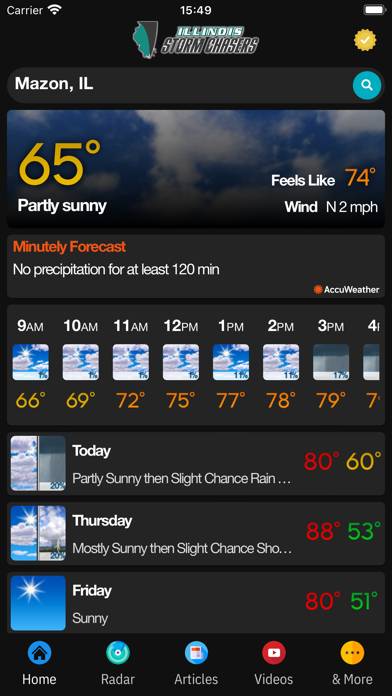The image displays a detailed weather interface for Illinois Storm Chasers. The page layout includes a black header with the text "Illinois Storm Chasers" and a golden verification tick on the right side, lending authenticity to the source. Below the header, there is a blue search bar displaying the text "Maison Isle" prominently. The primary section indicates the current weather as 65 degrees Fahrenheit and partly sunny, written in orange and white respectively, with a background of a blue sky adorned with high clouds. To the right, additional weather details specify it feels like 74 degrees with a wind speed of 2 miles per hour, and a forecast that notes no precipitation for the next 120 minutes, asserting the data's accuracy.

The hourly forecast spans from 9am to 4pm:
- 9am: 66 degrees
- 10am: 69 degrees
- 11am: 72 degrees
- 12pm: 75 degrees
- 1pm: 77 degrees
- 2pm: 78 degrees
- 3pm: 79 degrees
- 4pm: 79 degrees

A summary at the bottom of the image lists the daily forecast with high and low temperatures color-coded in red for highs and green/yellow for lows:
- Today: Partly sunny with a slight chance of rain, high of 80 degrees and low of 60 degrees.
- Tuesday: Mostly sunny with a slight chance of showers, high of 88 degrees and low of 53 degrees.
- Friday: Sunny with a high of 80 degrees and low of 50 degrees.

Navigational buttons line the bottom of the interface, providing quick access to Home, Radar, Articles, Videos, and more, enhancing user interaction and accessibility.